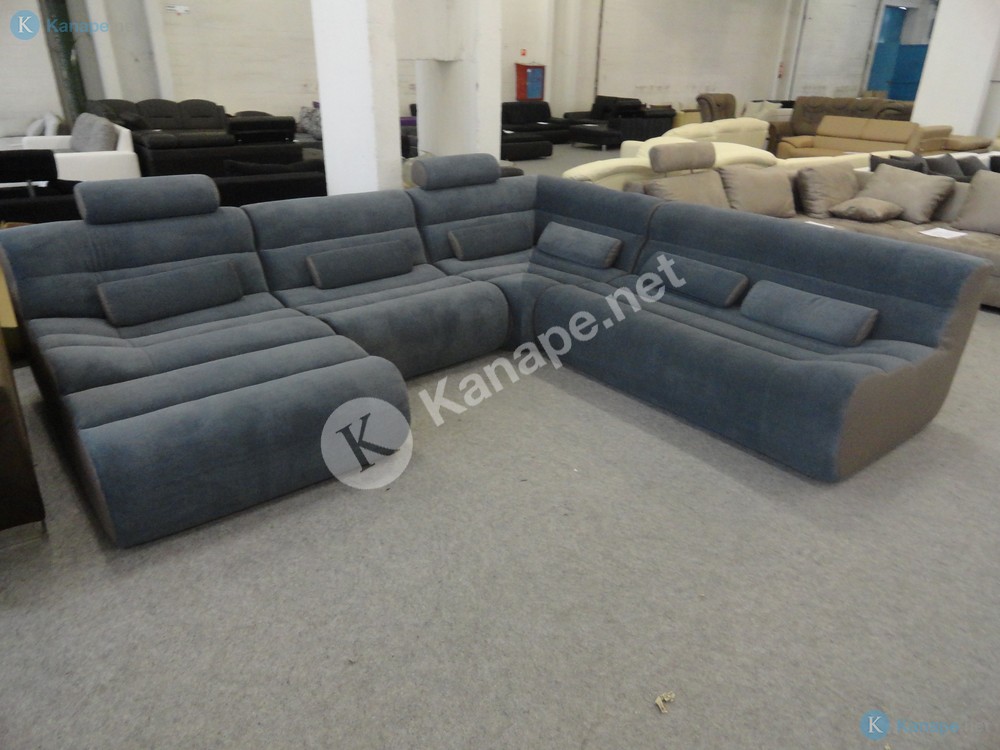This detailed photograph captures the interior of a large furniture store, clearly labeled with the watermark "K” in a circle alongside "K-A-N-A-P-E.net" in the center and lower right corner. The spacious showroom features a wide selection of sofas, including straight-line couches, sectionals, and wraparound models. The most prominently displayed sofa is a luxurious navy blue sectional with a chaise lounge, featuring a plush, velvety texture and cylindrical pillows adorning it, inviting comfort and relaxation.

Surrounding the main sofa, the diverse collection includes a beige couch, a cream-colored sofa, and several black couches strategically placed throughout the space. The spacious area also showcases multiple living room sets, complete with matching chairs and recliners. The room has a gray carpet that provides a neutral backdrop, and white support pillars are strategically positioned within the expansive space. Various colors of other couches, including khaki brown, gray, and white, are dotted around, illustrating the extensive variety available for purchase. The overall scene presents a well-organized display of home furnishings, perfectly suited for enhancing any living room.